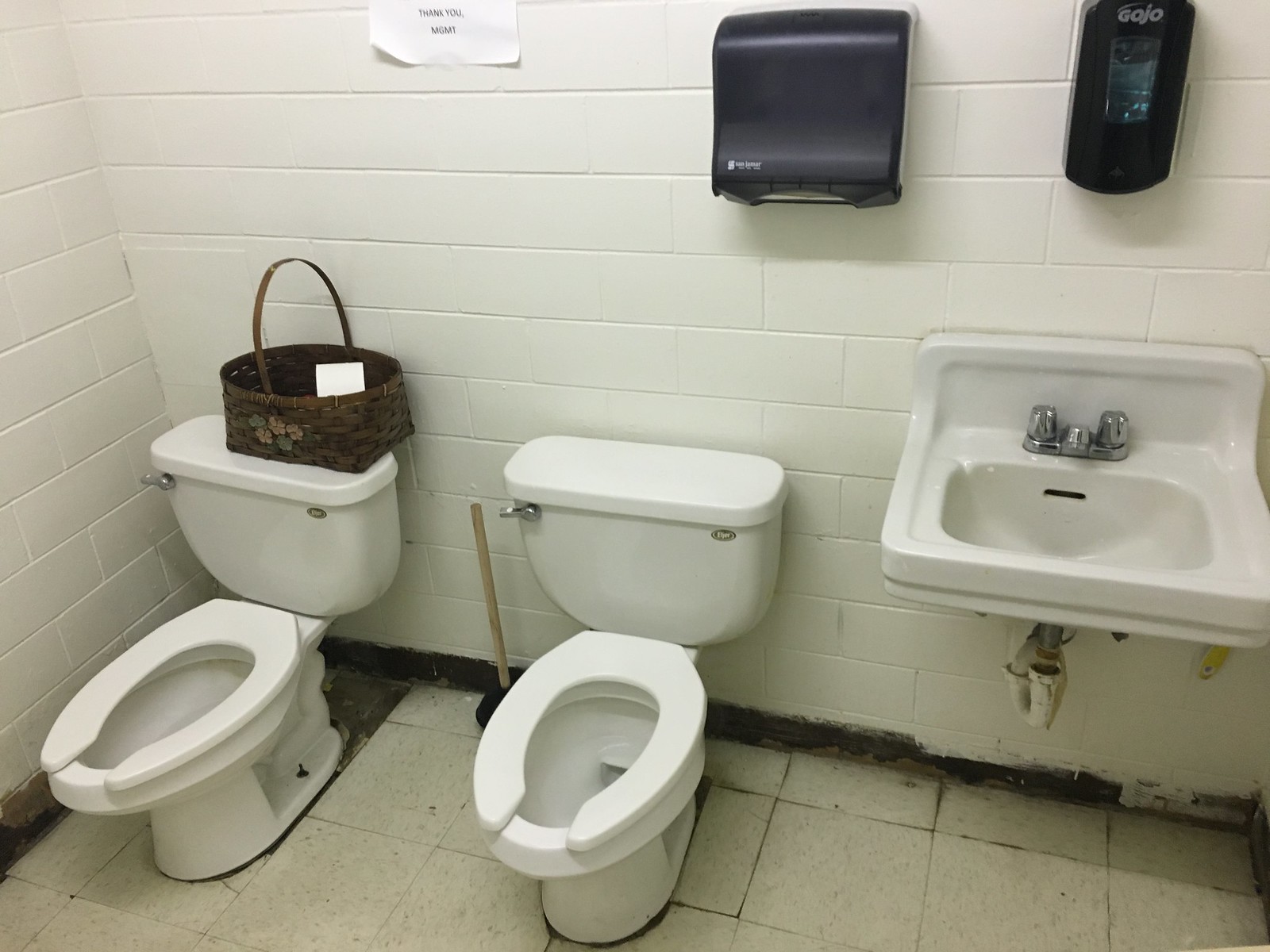This color photograph depicts a commercial public restroom with white painted brick walls and a mixture of white tiled and tan tiled floors. Dominating the center of the image are two side-by-side porcelain toilets, both equipped with open front seats but lacking lids. The toilet further to the left has a woven brown basket on top, possibly containing additional rolls of toilet paper. A black-handled plunger stands on the floor between the two toilets. Adjacent to the toilets on the right is a white porcelain sink with silver faucet handles, mounted on the wall. Above the sink, a black plastic soap dispenser is attached to the wall. To the left of the sink, a black plastic paper towel dispenser is fixed to the wall. There is also a sheet of white paper taped to the wall between the paper towel dispenser and the sink, bearing the message "Thank you, Management." The floor tiles appear dirty and soiled, particularly behind the toilets, highlighting distinct brown and black grime.